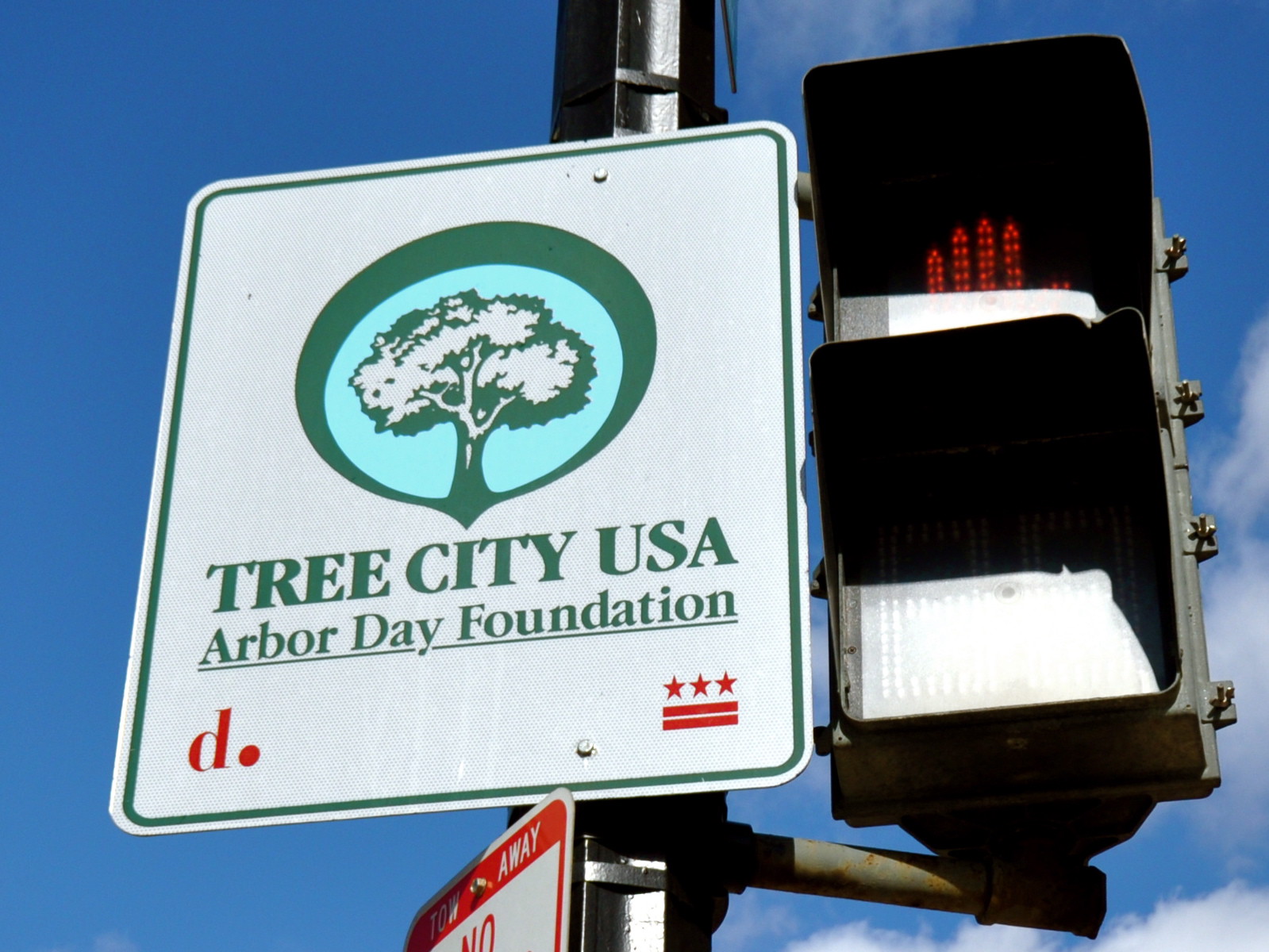This image captures a detailed view of a street sign and stoplight against a bright blue sky with a few transparent white clouds in the bottom left corner. The central black, shiny pole extends vertically through the middle of the frame. Mounted on the left side of the pole is a white rectangular sign with rounded corners and a green border. Dominating the sign is a green oval logo with a smaller blue oval inside it, featuring a green tree illustration. The sign prominently reads "Tree City USA" in bright green letters, with "Arbor Day Foundation" underlined beneath it. Adjacent to the sign on the right, there is a pedestrian streetlight with two lights. The top light flashes a red hand against a black cover, signaling to pedestrians. The streetlight is attached to a metal beam that projects outwards from the main pole, adding to the urban streetscape.